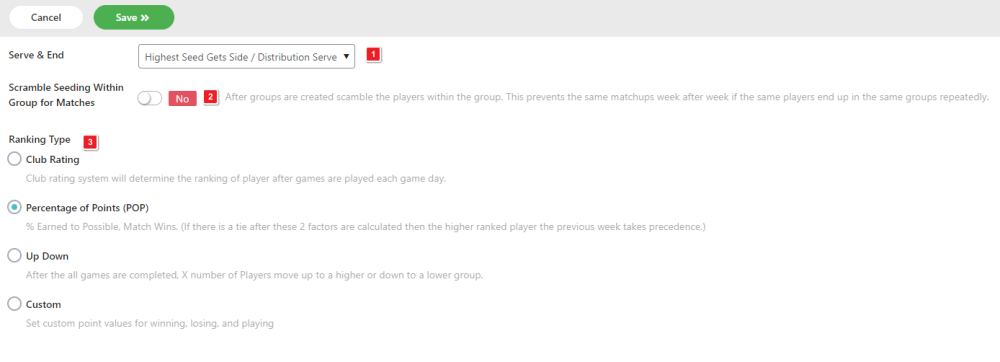The screenshot features a completely white background with a light purple rectangular header at the top. Within this header, there is a horizontally-aligned white oval on the left labeled "Cancel" in clear text. Adjacent to this is a green oval that reads "Save" in white text, accompanied by two right-pointing arrows.

Directly below the header, the text "Serve & End" is displayed prominently. To the right of this text is a white rectangular field containing the phrase "Highest seed gets side/distribution save," accompanied by a downward-pointing arrow, indicating a dropdown menu. A small red square bearing the number "1" is visible to the right of this rectangle.

Further down and to the left, the text "Scramble seeding within group for matches" is present, with a toggle switch to its right that is currently set to the "off" position. Next to this switch are two small red boxes: one labeled "No" and another labeled with the number "2."